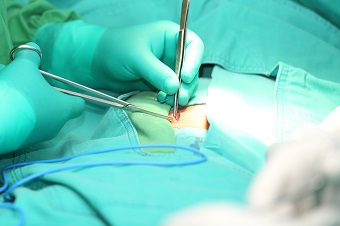In this close-up photo taken during surgery, the scene is dominated by the meticulous hands of a surgeon. The surgeon is donned in yellow scrubs and blue latex gloves, working diligently with stainless steel utensils, including tweezers in the left hand and a scissor-like instrument in the right. The patient is draped in a blue medical blanket, only exposing a small, focused area of skin through an opening in its center. Bright surgical lights shine down from above, providing the necessary illumination. Due to the tight framing, the number of assisting medical staff is indeterminable, and the exact nature of the surgical procedure remains unclear. The precision of the surgeon's actions is highlighted by the tools delicately manipulating the incision.